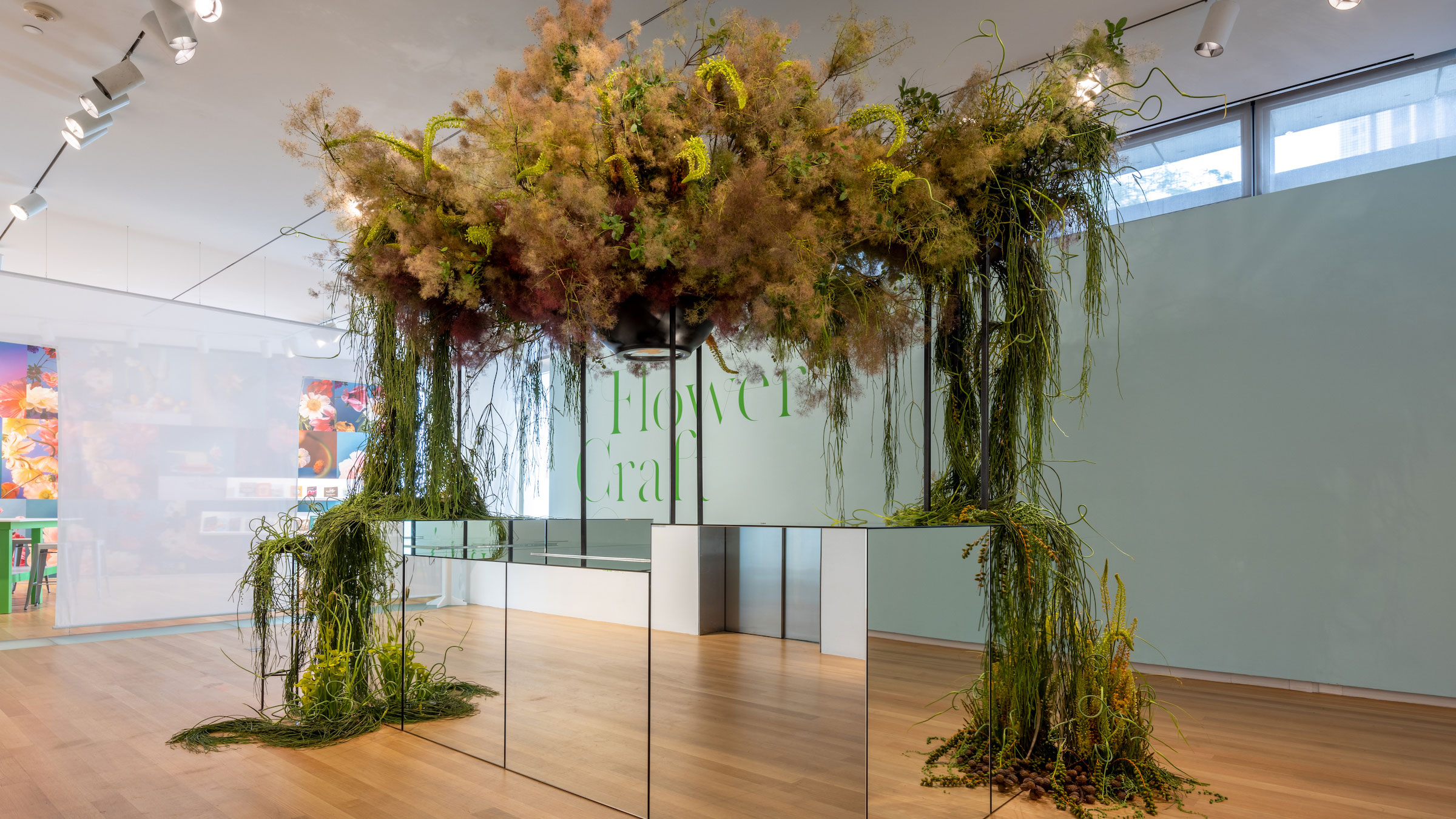The photograph is a landscape layout showcasing a museum interior with white walls and a smooth, light brown hardwood floor. The room is large and rectangular, featuring a white ceiling adorned with bright track lighting. At the center of the image is a prominent display consisting of stacked square mirror boxes, gleaming and reflective. Above this arrangement is an elaborate plant fixture, comprising lush greenery, beige and yellow floral elements, and green, thin moss-like strands hanging down. On the left wall, a collection of vibrant floral artwork can be seen, incorporating hues of pink, blue, yellow, and green. The overall setting is airy and well-lit, with small windows near the ceiling providing additional light.